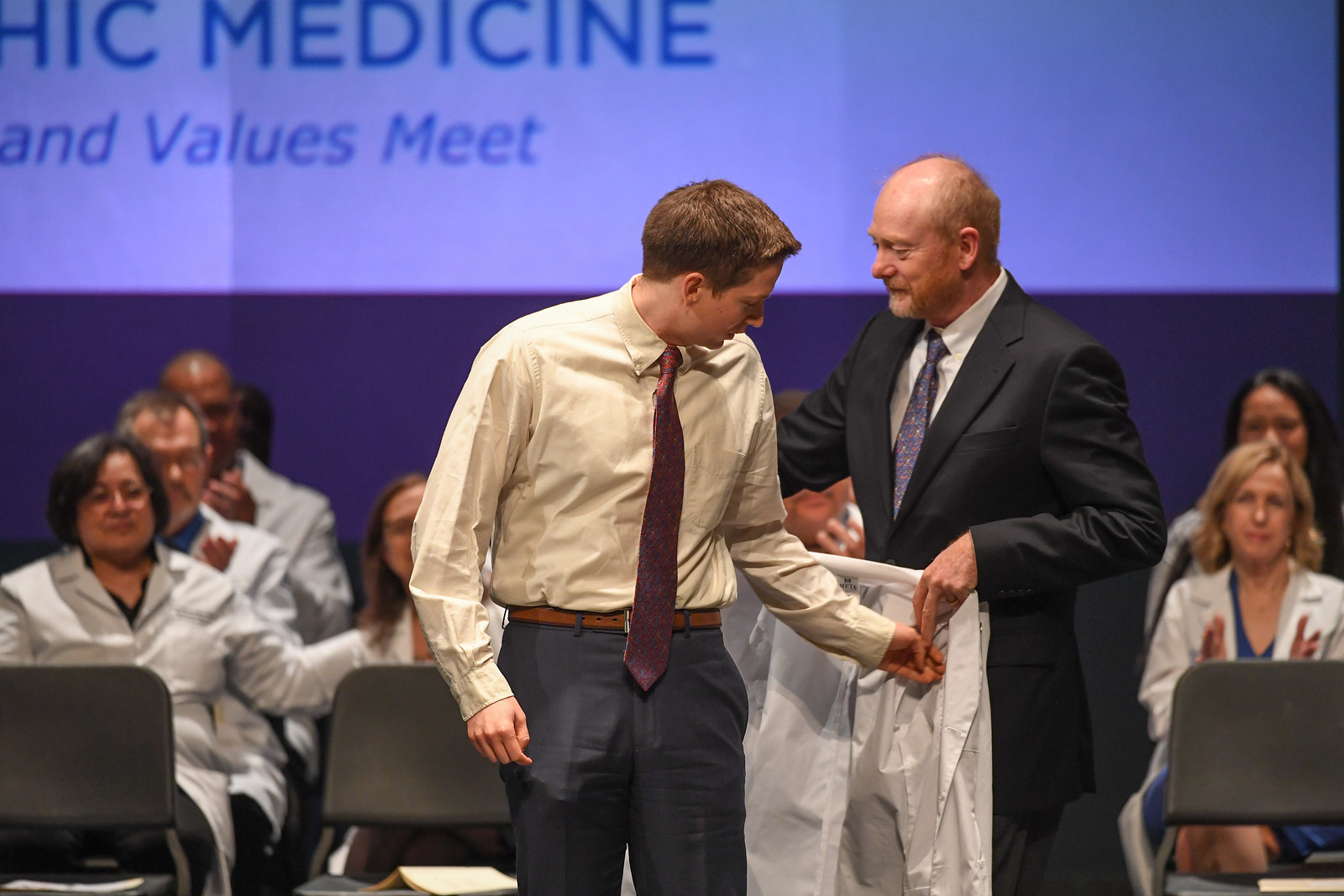The image depicts a graduation ceremony for new doctors, centered around a younger man in his mid to late 20s, who is receiving his white lab coat—a symbolic milestone in medical education. The young man, dressed in gray slacks, a tan shirt, and a burgundy tie, is slipping his arm into one sleeve of the coat, which is being held by an older gentleman, likely in his late 20s to early 30s, who is dressed in an off-white suit, gray slacks, and a dark red patterned tie. Behind them, rows of seated men and women, all clad in white lab coats, applaud the festive occasion. The background features a sign that reads "HIC Medicine and Values Meet," emphasizing the significance of the event. The older gentleman presenting the coat has a black suit, complemented by a white shirt and a purple tie. The scene is a heartwarming depiction of a pivotal moment in the young doctor's career.